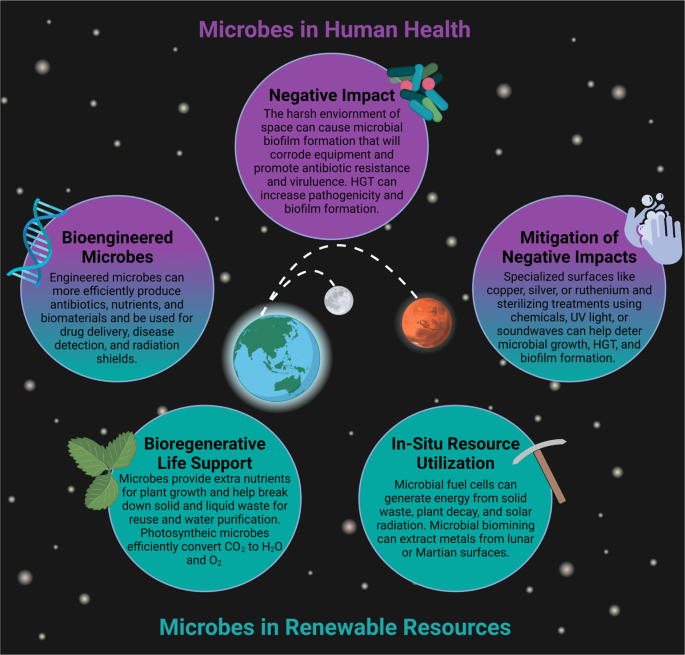The image depicts a scientific poster with the title "Microbes and Human Health" prominently displayed in purple lettering at the top. The poster is set against a black background dotted with stars. Central to the illustration is a blue and green Earth, flanked by Mars to its right and the Moon further to the right, all connected by dotted lines, suggesting a network.

Around the Earth are five evenly spaced, identical-sized circles, each with a heading in blue: 
1. "Negative Impact"
2. "Mitigation of Negative Impacts" (illustrated with two hands and soap bubbles)
3. "In-situ Resource Utilization"
4. "Bioregenerative Life Support"
5. "Bioengineered Microbes"

Each circle contains text explaining these topics. At the bottom of the poster, it reads "Microbes in Renewable Resources" in teal. The overarching theme of the diagram connects how microbes affect human health through various impacts, mitigation strategies, and their potential in resource utilization and bioengineering within the context of Earth, the Moon, and Mars.